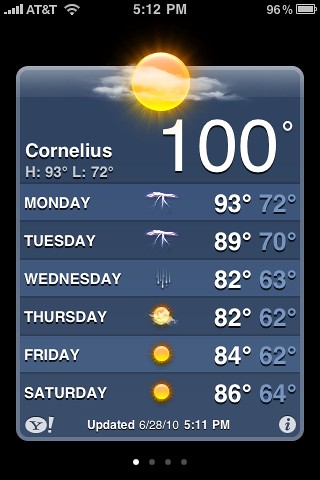The image depicts a detailed screenshot of a weather app on a cell phone, shown with an AT&T service logo at the top, including signal bars, a Wi-Fi indicator, and a battery icon at 96% at 5:12 PM. The primary weather information is displayed against a blue backdrop featuring a sun icon partially obscured by clouds. The location stated is Cornelius, with a current temperature of 100°F. Below this, a gray rectangular band provides detailed weather forecasts, showing a high of 93°F and a low of 72°F for Cornelius. 

The weekly forecast starts with Monday, showing a high of 93°F and a low of 72°F with a lightning bolt icon, indicating thunderstorms. Tuesday features similar thunderstorm graphics with temperatures of 89°F and 70°F. Wednesday displays a rain icon with temperatures of 82°F and 63°F. Thursday presents a partly sunny graphic, forecasting temperatures of 82°F and 62°F. Friday and Saturday are both represented by a full sun icon, predicting 84°F and 62°F, and 86°F and 64°F respectively.

The lower left corner of the image bears the Yahoo! logo and an exclamation mark. The bottom right corner contains a circular icon with the letter "i." Additionally, the bottom footer text reads, “updated 6/28/10, 5:11 PM.” The entire visual is encased within a black border, enhancing the clear visibility of white and blue text against the blue and gray backgrounds.